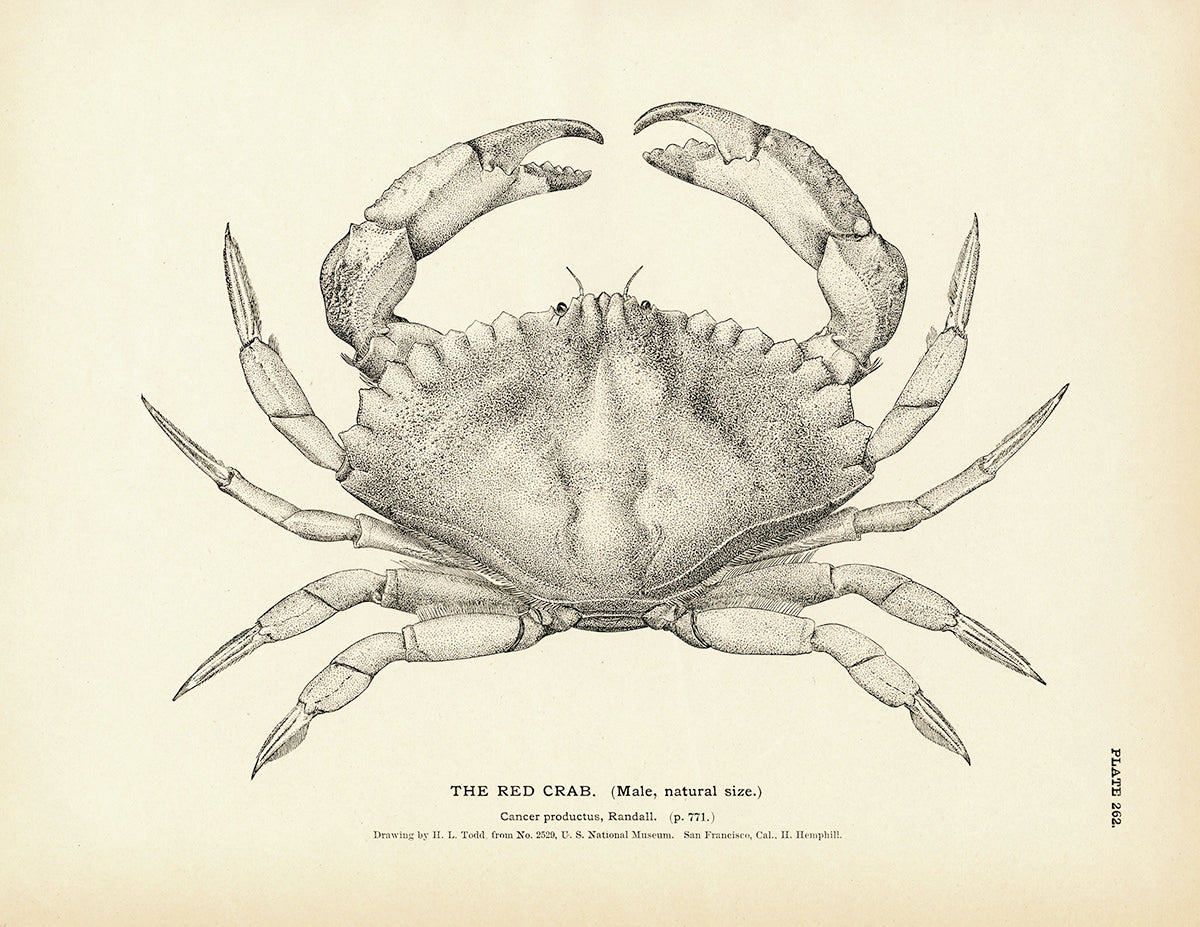This detailed artwork depicts a black and white illustration of a crab, known as "The Red Crab (Male), Natural Size, Cancer Productus, Randall." The drawing, executed by H. L. Todd, is labeled as originating from the U.S. National Museum, San Francisco, California, catalog number 2529, and is credited to H. Hemphill. The image is presented on an aged, parchment-like piece of paper with a weathered appearance, exhibiting darker tan edges that gradually transition to a lighter beige center. The crab illustration shows a top view, detailing its flat, serrated carapace and short legs, with two prominent pincers in front and eight legs fanning out from beneath. The uppermost legs curve upwards, while the bottom legs extend slightly downward. The illustration is highly detailed, reminiscent of a stippling technique, and includes textual notations such as "Plate 262" oriented vertically on the bottom right, and a descriptive caption beneath the crab reading "The Red Crab (Male), Natural Size, Cancer Productus, Randall, page 771, drawing by H.L. Todd from number 2529 U.S. National Museum, San Francisco, California, H. Hemphill."